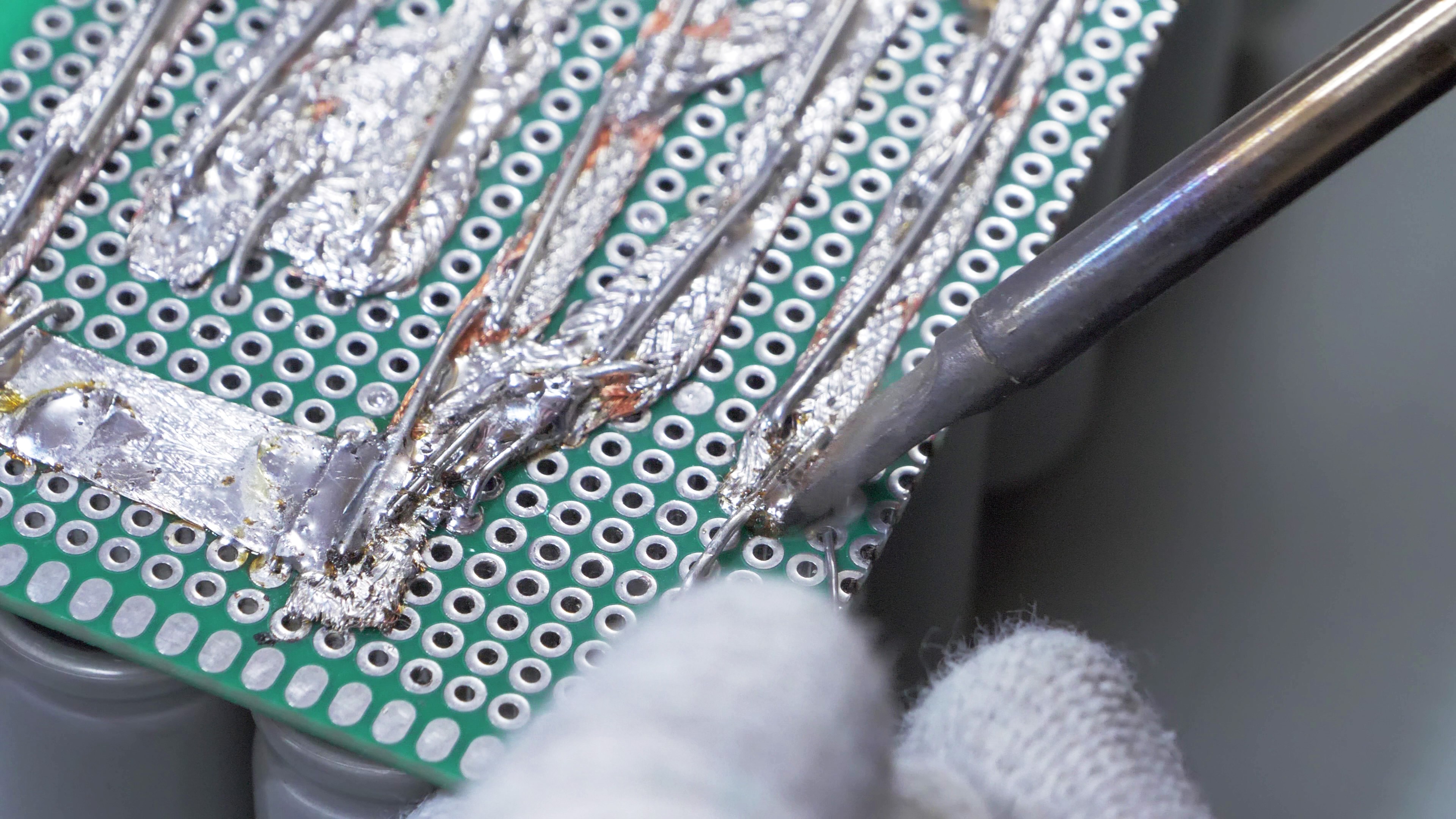The photograph captures a close-up view of a green motherboard being soldered, set against a blurry gray background. Dominating the middle to upper left side of the image is a partially visible green rectangular or square component, perforated with numerous tiny circles and partially covered in foil, from which a mesh of silver wires extends. In the upper right corner, a soldering iron, resembling a pen with a gold top and silver bottom, makes contact with the wires and foil. The person performing the soldering is wearing white, fuzzy gloves, and their technique appears exceedingly messy, with visible rust stains and yellow liquid pooling at one end of the chipset. No text is present, and the color scheme includes shades of green, brown, silver, gray, white, and black.